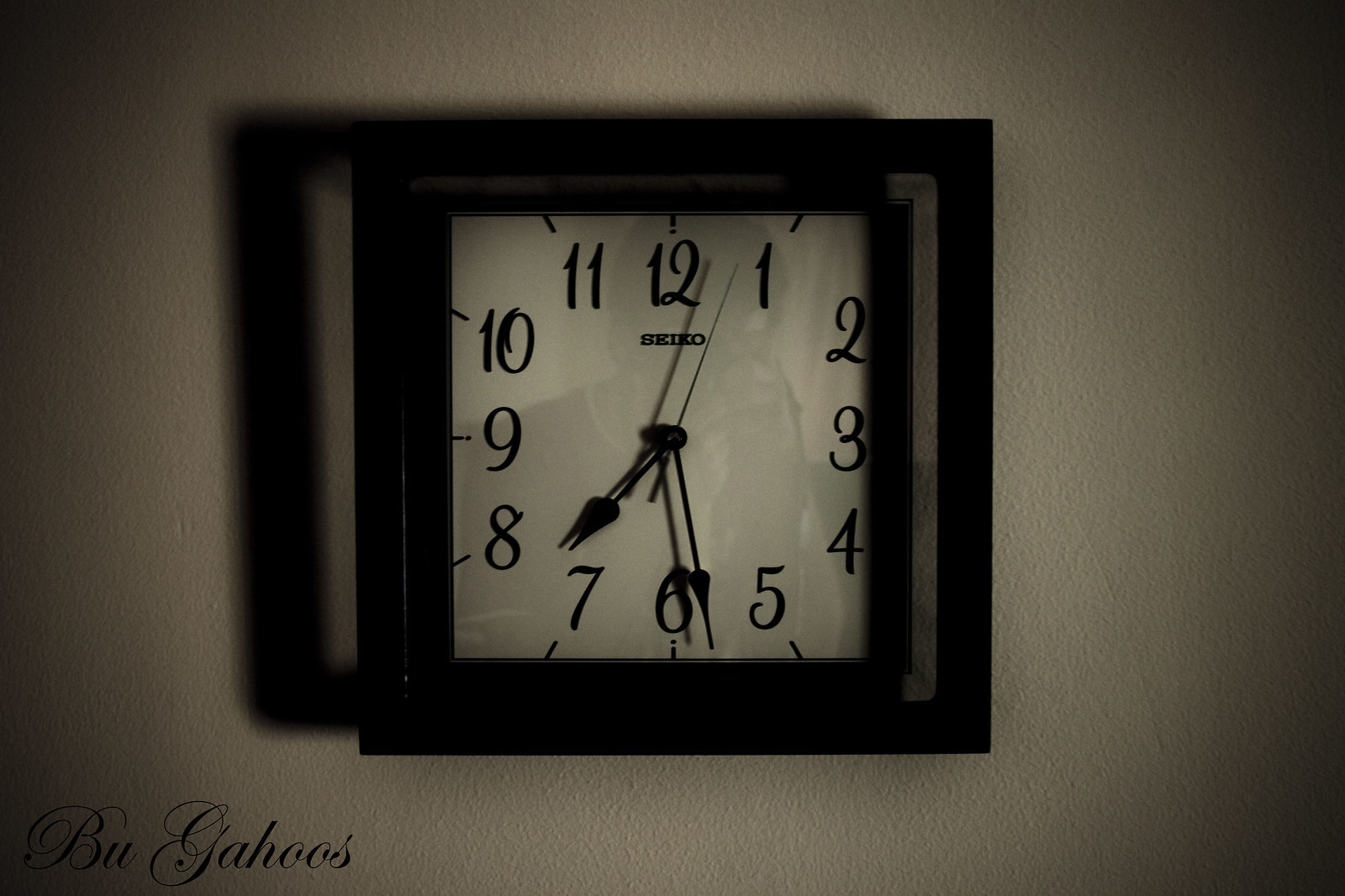This photograph showcases a square clock mounted on a white wall. The edges of the image on both the right and left sides have a subtle gray-shaded effect, framing the central composition. The clock itself features a sleek black frame that sharply contrasts with its white face. Large, black numerals mark the hours, although the numbers two, three, and four fall partially out of view due to cropping or shadow. The clock lacks minute markers, allowing the bold hour numerals to stand out. The center of the clock face holds a black circular hub from which the hands extend. Both the hour and minute hands are black and adorned with teardrop-shaped tips. A delicate gray second hand completes the ensemble, poised to indicate the passing moments. The time displayed is precisely 7:28.